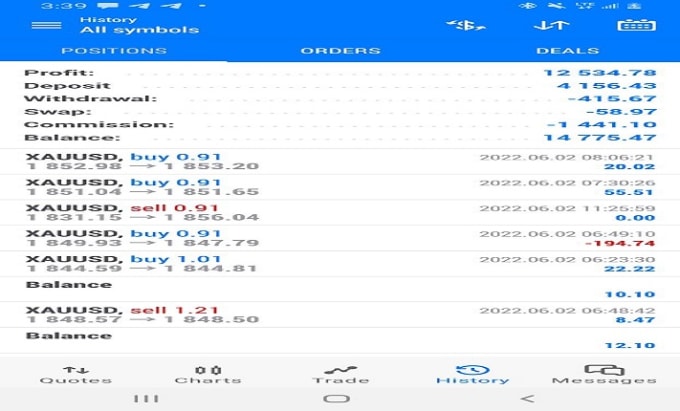A detailed widescreen screenshot of a mobile trading platform interface, featuring a somewhat stretched and zoomed-in display. The main section of the screen presents a summary of financial activities, including profit, deposits, withdrawals, swaps, commissions, and balance. The figures listed are as follows:

- **Profit:** $12,534.78
- **Deposit:** $4,156.43
- **Withdrawal:** -$415.67
- **Swap:** $58.97
- **Commission:** -$1,441.10
- **Balance:** $14,775.47

The trading instruments appear focused on **XAUUSD**, indicating trading activities involving gold versus the US dollar. These activities are detailed in a list format beneath the financial summary.

The interface has a clean, white background with balance numbers displayed in blue, and negative figures shown in red. The top portion of the screen includes navigational tabs labeled **History, Positions, Orders, and Deals**. Meanwhile, the bottom of the screen features secondary navigation tabs labeled **Quotes, Charts, Trade, History, and Messages**. 

Despite the layout, the specific trading platform isn't immediately identifiable due to an absence of a discernible logo, though the blue color scheme hints it might be something similar to Coinbase.